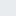A completely light gray square with no distinguishable features. The image appears to be devoid of any content, possibly due to a loading error.